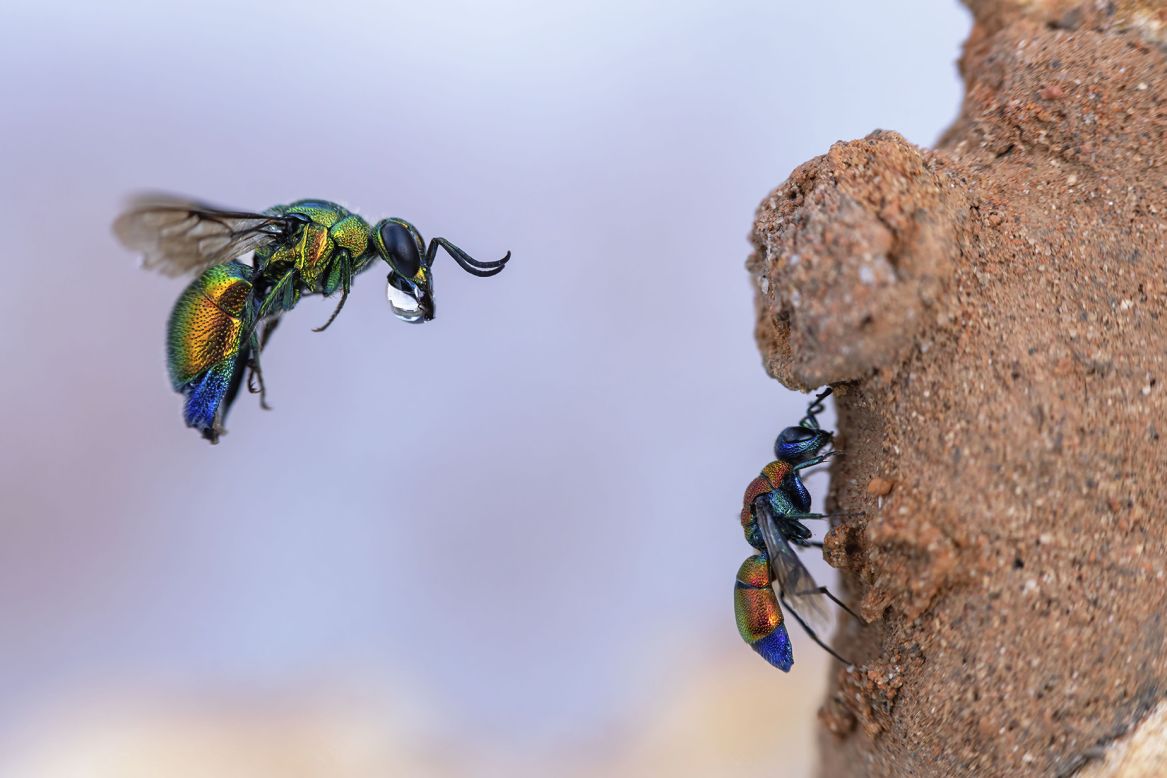In this vividly colorful close-up photograph, two brilliantly colored winged insects, possibly a type of flies, are the focal point. The background is a blur of blue with faint cloud-like suggestions, making the insects and the scene's main elements stand out sharply. On the right side of the image, one insect is perched atop a vertical mound that appears to be made of sand or dirt, constructed in a way that could resemble their nest. This insect dazzles with metallic shades of blue, gold, and green, with particularly striking highlights on its thorax, which appears more red. On the left, the second insect is captured in mid-flight, headed towards the same structure. It carries a tiny drop of water in its mouth, which is quite visible against the insect's equally vivid coloring. This flying insect shares the same vibrant palette as the perched one, though its thorax is more green, likely due to the angle of light. Both insects have long, noticeable antennae and translucent wings, adding to their stunning appearance.